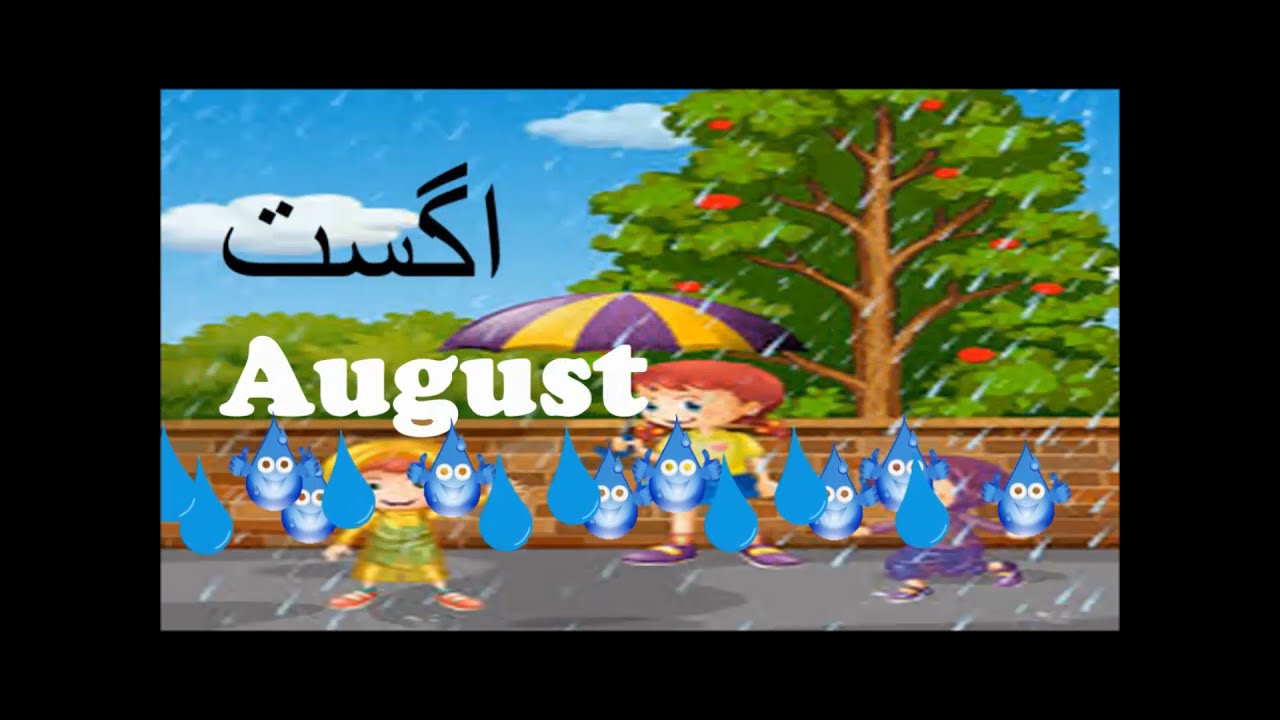The image appears to be a colorful, digitally created scene, likely a screenshot from a video or a video game, showcasing a charming rainy day. The scene features three children, rendered in a nostalgic, late 90s to early 2000s cartoonish video game style. 

In the center, a young girl with red hair stands holding a purple and yellow striped umbrella. She is dressed in a yellow shirt, blue shorts, orange socks, and purple sandals. To her right is a young boy with orange hair, wearing a yellow raincoat and blue socks with orange shoes. The third child, on the far right, has orange hair under a purple hoodie, paired with purple shorts and shoes.

They are standing on a sidewalk in front of a brown brick wall that reaches up to the children's heads. Behind the wall, a large tree with green leaves and red apples is visible, and parts of a blue sky with white clouds peek through. A green bush can be seen beside the tree. 

Adding to the whimsical atmosphere, several cartoon raindrops with googly eyes and smiling faces are scattered across the scene. The raindrops vary in size, with some larger ones taking a prominent place in the foreground, and smaller ones appearing to splash playfully at angles.

A thick black border frames the image horizontally, being thinner at the top and bottom. In the upper middle section, the word "August" is boldly displayed in white letters. Above it, there is text in Arabic script, adding an additional layer of cultural detail to the composition.